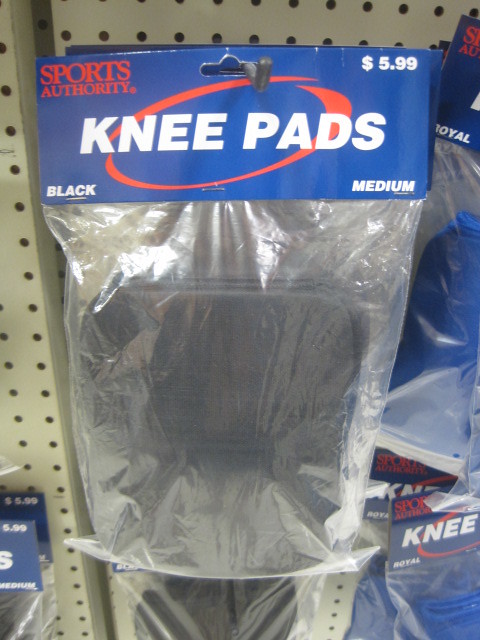This image showcases a package of black knee pads prominently displayed on a metal shelf with holes, likely in a store. The knee pads are enclosed in a transparent plastic bag with a sturdy cardboard top, creating a secure package. The cardboard top features a predominantly blue design with key details highlighted: at the top left, "Sports Authority" is written in red text, while the top right corner displays the price "$5.99." Centered across the front of the packaging, in large white text, is the label "Knee Pads." At the bottom, further details specify "Black" and "Medium" in white text. Surrounding this centrally featured package, other knee pad products are partially visible, enhancing the retail environment context of the photograph.